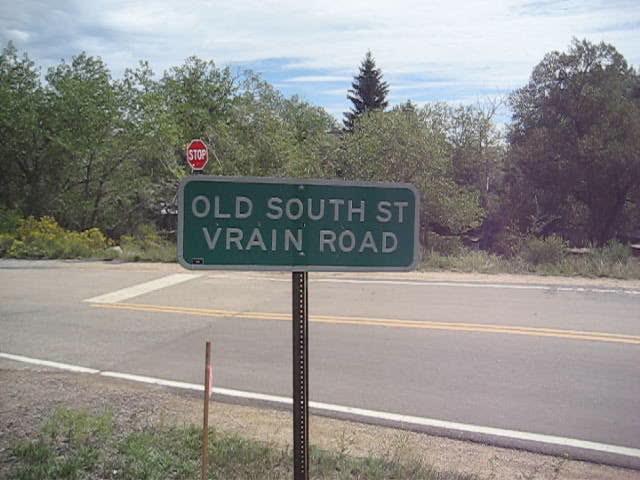A horizontal photograph captures a serene country scene, dominated by a two-lane highway that runs diagonally from the lower right corner towards the left center of the frame. This rural road, flanked by patches of grass, comes to a halt at a prominent stop sign positioned at the center of the image. Just below the red stop sign, a green street sign with a white border is mounted on a robust metal pole, emblazoned with the names "Old South Street" and "V-R-A-I-N Road" in bold, uppercase white letters. Adjacent to the signpost, a short yellow post stands on the left side. The road is surrounded by an expanse of lush greenery, with trees sprawling across the background and a possible pond situated towards the center right. The sky above is a vibrant blue, adorned with a generous scattering of white clouds, lending a peaceful ambiance to the scenic countryside vista.